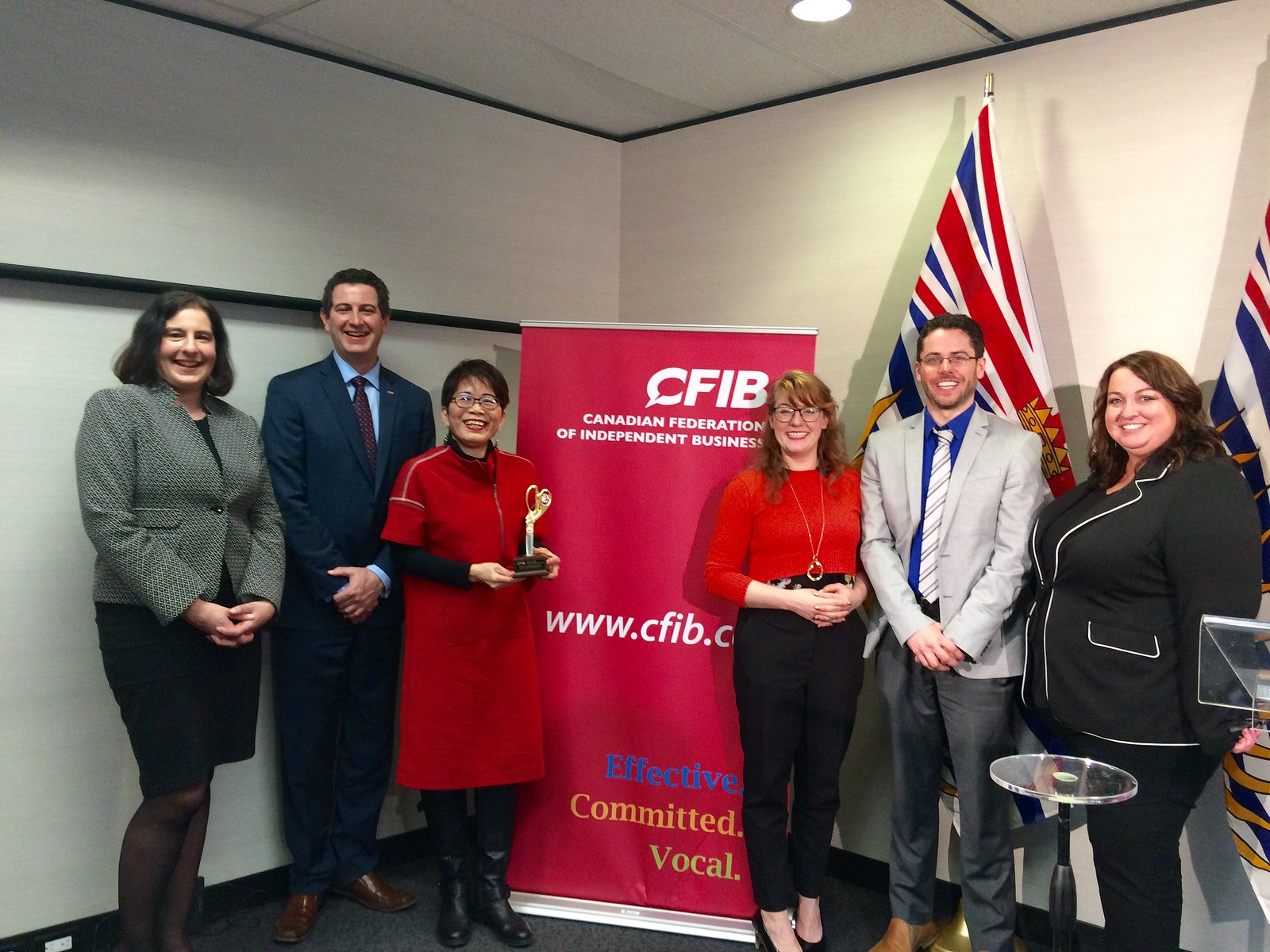In this indoor photograph, six individuals pose in a corner of a beige-walled room, flanked by two Canadian flags and a clear plexiglass podium. At the center of the image, a red floor banner stands prominently, displaying the text "CFIB, Canadian Federation of Independent Business, www.cfib.com, effective committed vocal" in white, blue, yellow, and green lettering. On the left side, a woman in a black skirt, black tights, and a tweed jacket stands beside a man dressed in a blue suit, light blue shirt, and tie. Next to him is a woman in a red dress and black boots, holding an award shaped like a golden pair of scissors. On the right side of the banner, a woman wearing black pants, black heels, a red shirt, and glasses stands next to a man in dark slacks, a light gray suit jacket, blue shirt, striped tie, and glasses. To the far right, a woman in a black suit with white piping completes the group. All individuals are attired in business formal or business casual attire, exemplifying a professional setting.